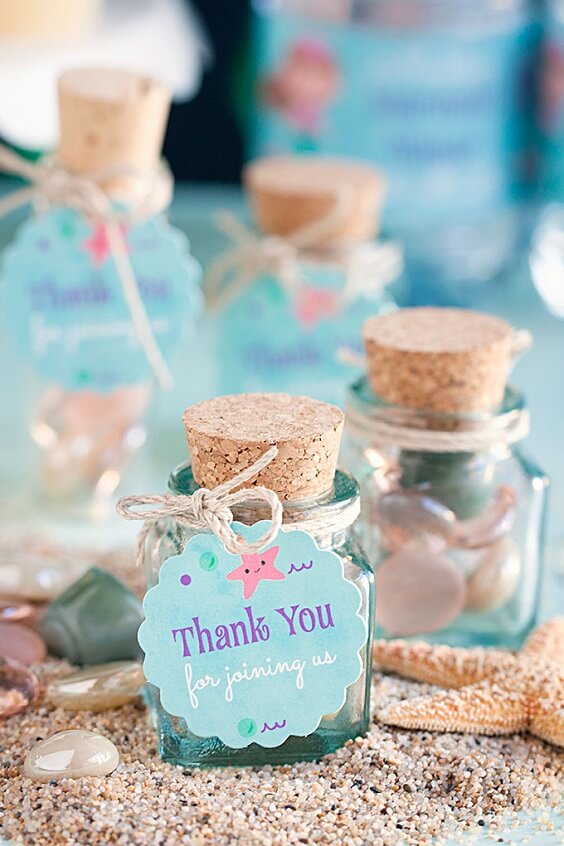The image features a collection of tiny, transparent jars, each capped with a small, brown cork. The jar in the foreground stands out prominently with a light blue, curve-edged tag that reads "Thank you" in purple, and "for joining us" in white beneath it. Adorning the tag is a playful, cartoonish pink starfish with two eyes and a smiley face. The tag is tied with a white rope. Inside this jar, the contents are not visible, but to the back right, another jar appears to contain decorative stones. The jars in the background are progressively more blurred. All these jars are situated on a sandy surface scattered with similar decorative rocks, completing a charming and whimsical scene.